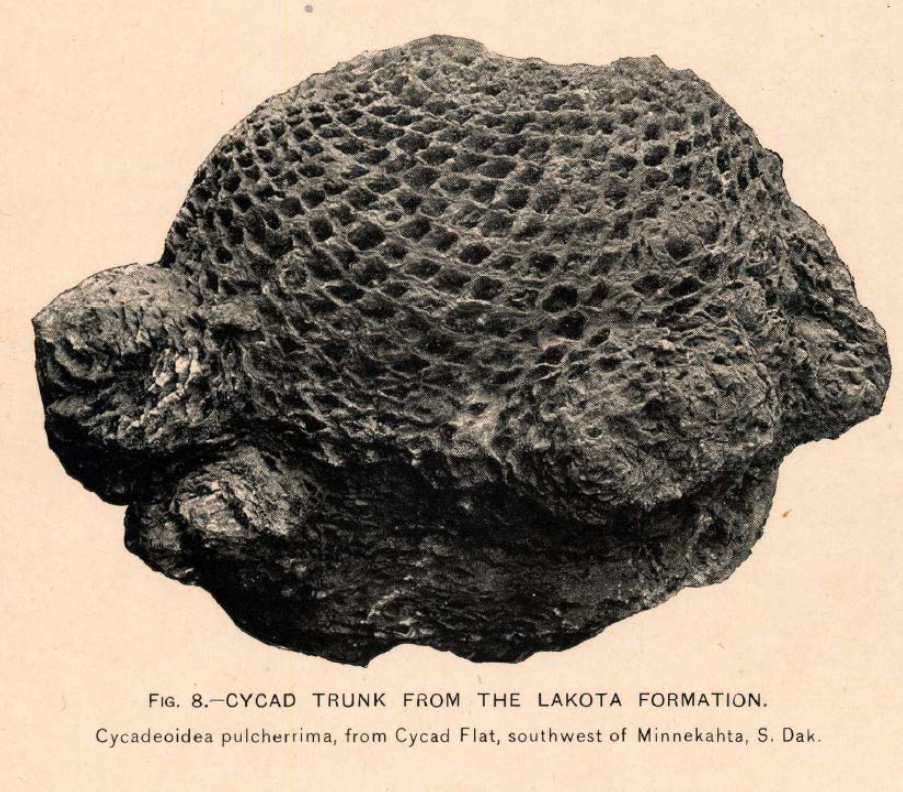This detailed photograph displays a unique, dark charcoal gray rock formation resembling a petrified honeycomb. The artifact, which has a porous top with a distinct diamond-patterned honeycomb structure, gradually transitions to a more solid base. The object is almost spherical and evokes the shape of a turtle, with the honeycomb section reminiscent of a turtle's shell. It is showcased on a pale tangerine background with black lettering at the bottom that reads: "FIG. 8, CYCAD TRUNK FROM THE LAKOTA FORMATION." Beneath this, in Latin, "Cycadoidea Pokornyi" is noted, alongside its geographical origin: "From Cycad Flat, southwest of Minnecotah, South Dakota."